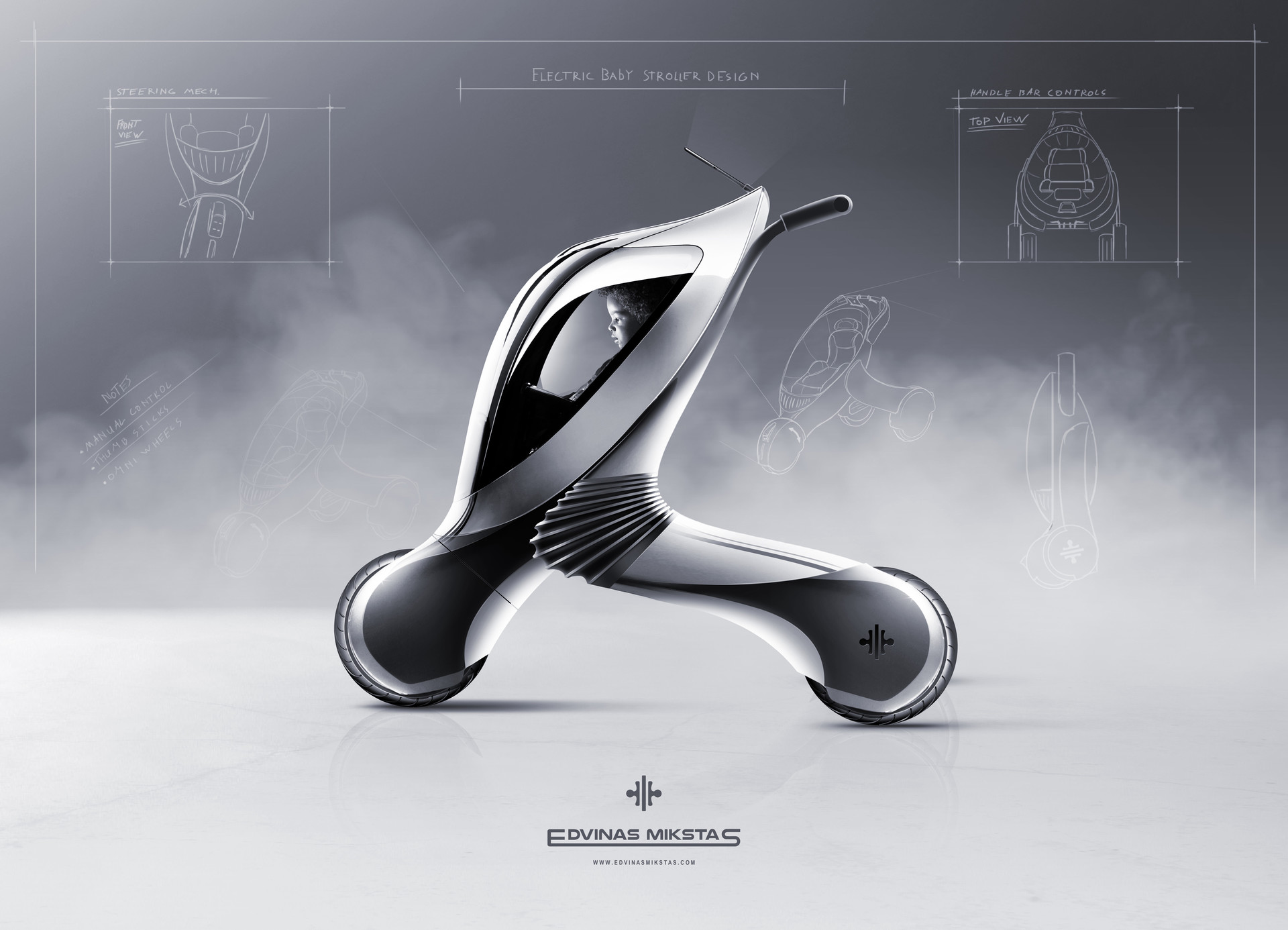The image presents a sophisticated, futuristic prototype of an electric baby stroller. The scene is primarily grayscale, accentuating a sleek, silver-chrome device at the forefront. This design features a central, pod-like cab with a curved, eye-shaped window through which a child with curly hair and dark skin is visible, illuminated gently by the ambient light. The cab is supported by two protrusions; the one in front mimics a tire and extends diagonally beneath the pod, while the rear one, longer and more angled, ensures stability. Both supports are equipped with wheels. Above the device, in delicate white lettering, the title "Electric Baby Stroller Design" is displayed, accompanied by artist renderings in the corners and various notes such as "manual control" and "turbo sticks." The background of the image is a misty gray with a subtle fog-like texture, enhancing the contrast of the precise, white line drawings that demonstrate the stroller's functionalities, including a top view revealing the seat, a detailed side view, and annotations about its foldable design. This stylish and potentially high-cost innovation combines advanced technology with modern aesthetic principles.